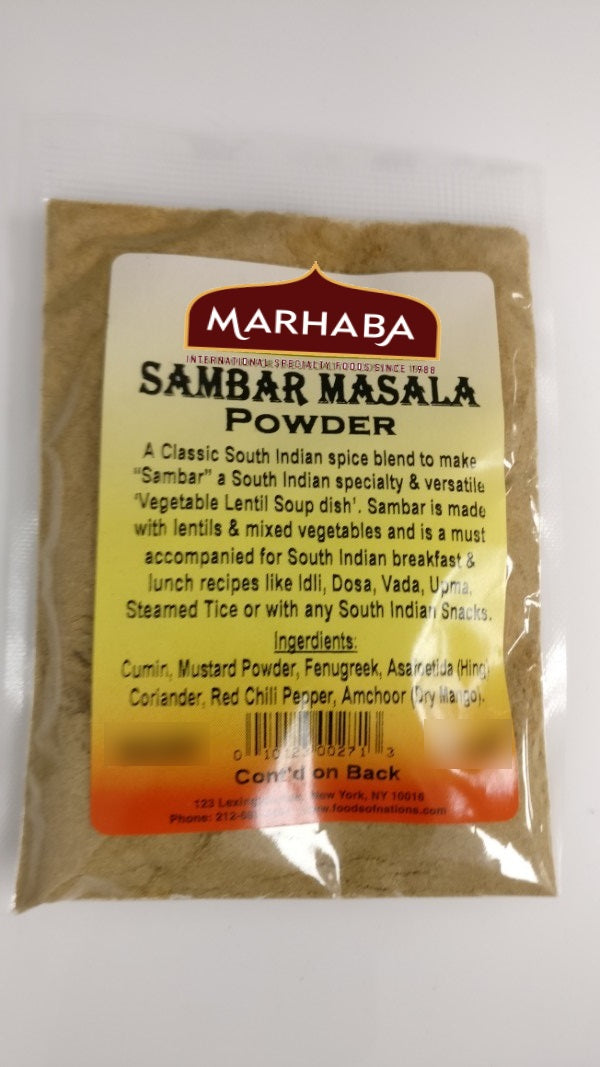This is a detailed photograph of a package of Marhaba Sambar Masala Powder, a classic South Indian spice blend essential for preparing sambar—a versatile and traditional vegetable lentil soup dish. Sambar is a staple in South Indian cuisine, enjoyed for breakfast and lunch alongside dishes such as idli, dosa, vada, upma, steamed rice, and a variety of snacks. The package lists ingredients including cumin, mustard powder, fenugreek, coriander, red chili pepper, amchur (dried mango), and hing (asafoetida). The powder itself appears light brown and is wrapped in clear plastic, featuring a barcode at the bottom. The package indicates it is distributed from New York and includes a contact phone number.